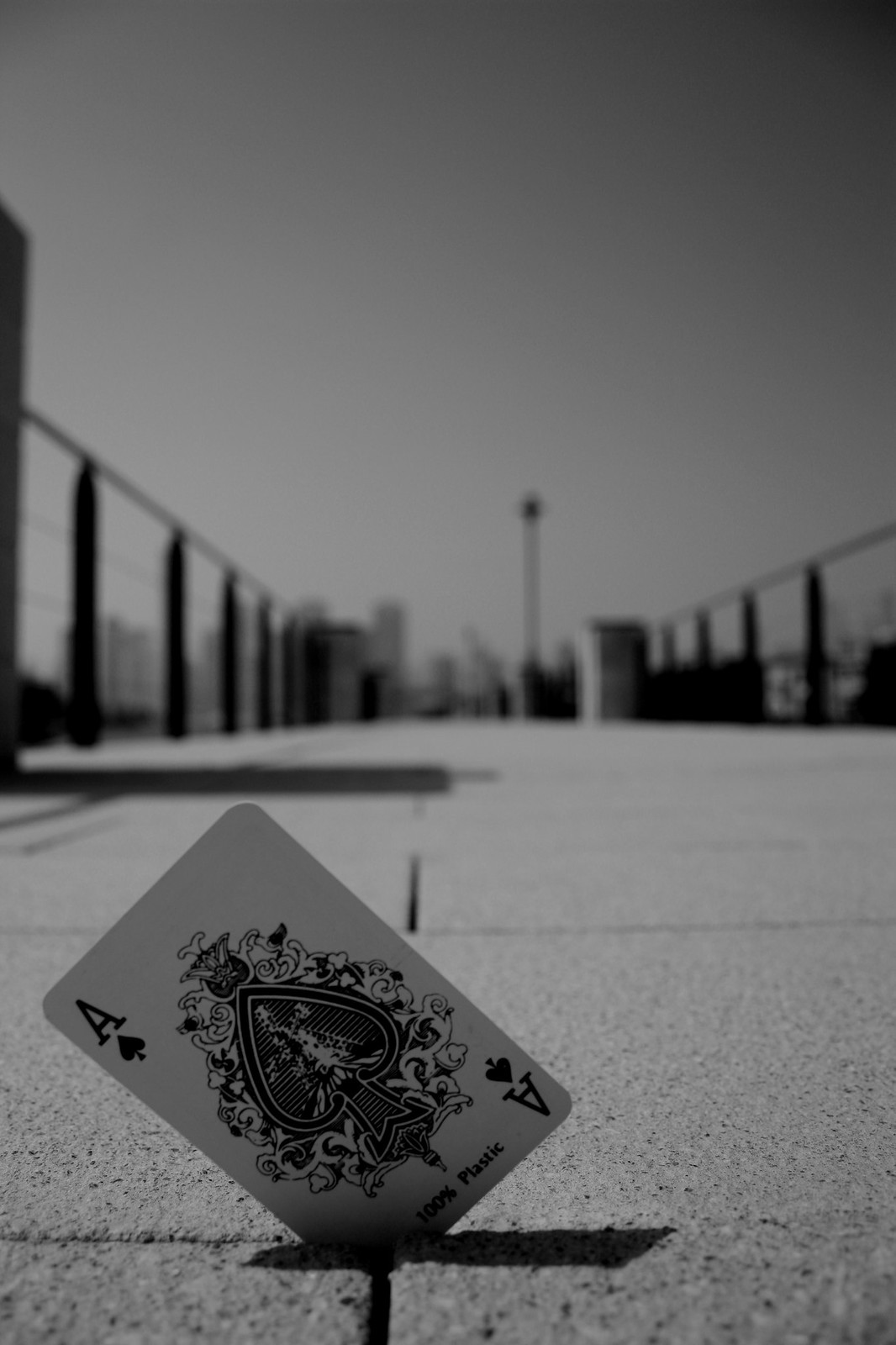This evocative black-and-white photograph, accentuated with subtle hints of gray for an artistic effect, captures an intriguing urban scene. The image, oriented in portrait mode and approximately twice as tall as it is wide, is set against a minimalist white background that emphasizes its elements.

In the foreground, a detailed Ace of Spades playing card, labeled "100% plastic" at the bottom, lies conspicuously in a sidewalk crack. The central spade is intricately adorned with elaborate designs, drawing immediate attention. The card anchors the scene, situated among the silac tiles of the walking area, suggesting it might be part of a bridge or elevated walkway.

High walls flank both sides of the walkway, leading the eye towards the distant cityscape visible in the background. Vertical and horizontal cracks and lines in the pavement delineate individual blocks, adding texture to the photo. In the distance, a needle-like tower pierces the sky, flanked by pillars lining the edges of the walkway, enhancing the sense of depth and perspective. The juxtaposition of the singular playing card against the expansive urban backdrop invites viewers to ponder its symbolic significance within the metropolitan environment.